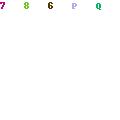In the image, we observe a screenshot of a website displayed on a computer screen. At the top of the browser, a gray navigation bar is visible, featuring a blue back arrow, a faded blue forward arrow, a bookmark icon, and a gray search bar with a white lock symbol, indicating a secure connection. The search bar displays the URL: "lifetime.bksblive2.co.uk". Adjacent to the search bar are the refresh and download icons, along with a blue plus icon for opening new tabs.

Multiple browser tabs are open. The first tab is titled "Buy HP Pavilion 14," and the second tab, which is currently active, is labeled "BKSB Assessment Player." 

Within the active tab, a blue banner dominates the top section, reiterating the title of the webpage: "BKSB English Initial Assessment." The user is currently on question 2 of the assessment. Just below the banner lies a navigation bar that includes a house icon and a circular icon that might represent a user profile or additional settings.

The main content area instructs the user to "Select the correct answers." The task involves choosing the correct words from the dropdown options provided below. A lengthy paragraph is present, containing two dropdown boxes. The user has already selected "although" for the first dropdown box and appears to be in the process of selecting an option for the second dropdown box.